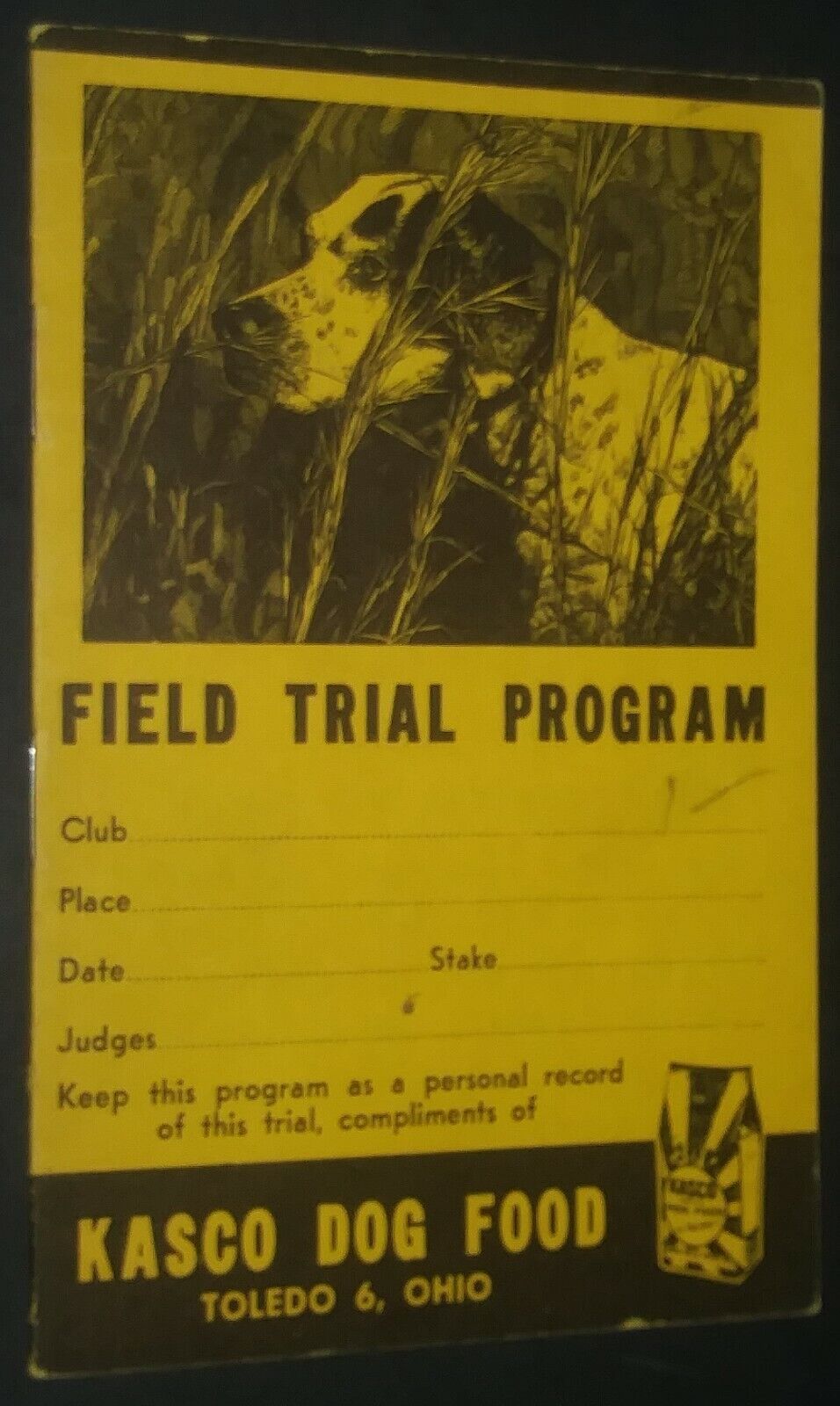This photograph showcases a vintage, yellow-and-black field trial program cover. Dominating the top half of the program is a detailed illustration of a Dalmatian-like dog, featuring floppy ears hanging by its sides, white fur adorned with dark spots, and set against a backdrop of tall grass. Directly beneath this, in bold black text, it reads "Field Trial Program." Below this title is a customizable section intended to record event details, labeled sequentially as "Club," "Place," "Date," "Stake," and "Judges," each with space for entries, though none are currently filled out. Further down, a message instructs, "Keep this program as a personal record of this trial. Compliments of," followed by a black banner displaying "Casco Dog Food, Toledo 6, Ohio" in white letters. In the bottom right, there is a low-resolution, slightly blurry photograph of a bag of Casco dog food.